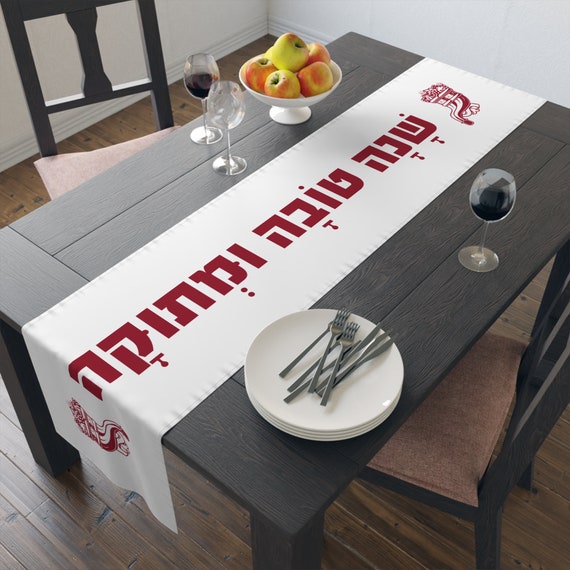This image captures an aerial perspective of a dining setup on a dark brown wooden table adorned with a white embroidered banner featuring red lettering, possibly in a Middle Eastern script. The table, situated in a kitchen-like area with white walls and a light wooden floor, is designed for four people, evidenced by the four white plates accompanied by silverware. The table's center is decorated with three wine glasses; one is empty, while the other two are half-filled with red wine. Near the glasses, a white bowl brimming with apples adds a touch of freshness. The chairs, featuring light tan cushions without armrests, are slightly pulled out at an angle. The soft, pastel lighting enhances the inviting appearance of the scene, making it an appetizing and cozy setup.